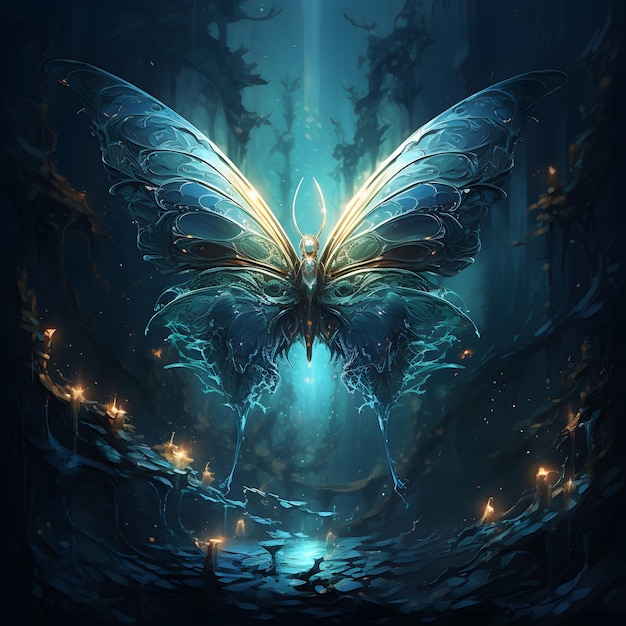The image depicts a fantastical scene centering around a large, ethereal butterfly that dominates the composition. This butterfly, or butterfly-inspired creature, boasts shimmering blue and green wings with intricate golden strands running throughout, creating a fluid, almost flame-like or water-like effect at the wavy ends of the wings. Each side features two distinct wing sections typical of both butterflies and moths, with the bottom sections tapering into long, tail-like appendages that nearly touch the ground. The butterfly's body is golden and elegant, complemented by long, elaborate antennae.

Set against an aqua blue and dark backdrop that deepens towards the edges, the scene is awash with varying shades of blues, blacks, and hints of gold, contributing to its mystical ambience. The background seems to merge elements of a mystical woodland and a cave, highlighted by bright, floaty lights and delicate fires burning atop blue-hued plants and wooden posts at the bottom. Scattered stones enhance the enchanting narrative of the image, all of which create an overall dark yet fantastically illuminated tableau.